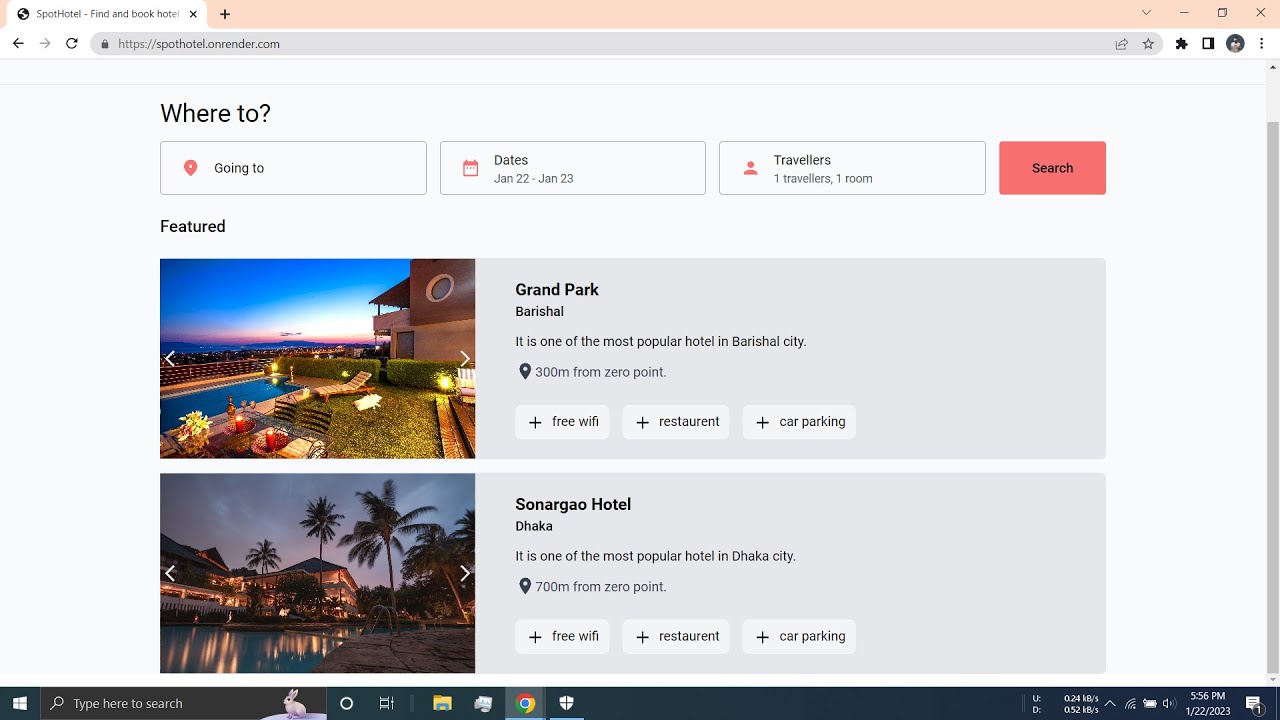The image shows a webpage open in a Google Chrome browser with a peach-colored header at the top. The left side of the browser tab displays a gray globe icon accompanying dark gray text that reads "SpotHotel - Find and Book Hotels," though the text is partially cut off. To the left of the URL bar, there are back and forward navigation buttons, where the forward button is disabled, indicated by its light gray color. Next to these is a dark gray refresh button.

The URL bar contains "https://spothotel.onrender.com," and beneath it, the page transitions to a light gray background. A faint border serves as a divider at the top. In the upper left corner, bold black text poses the question, "Where to?" Below this prompt, there are three interactive fields:

1. The first field, marked by a red map pin icon, is labeled "Going to" in black text.
2. The second field, adjacent to it, features a red calendar icon labeled "Dates" in black text, with smaller gray text below indicating "Jan 22 - Jan 23."
3. The third field, having a red silhouette of a user, is labeled "Travelers" in black text, with smaller gray text beneath stating "1 traveler, 1 room."

To the right of these fields, there is a red rectangular search button with bold, black text that reads "Search."